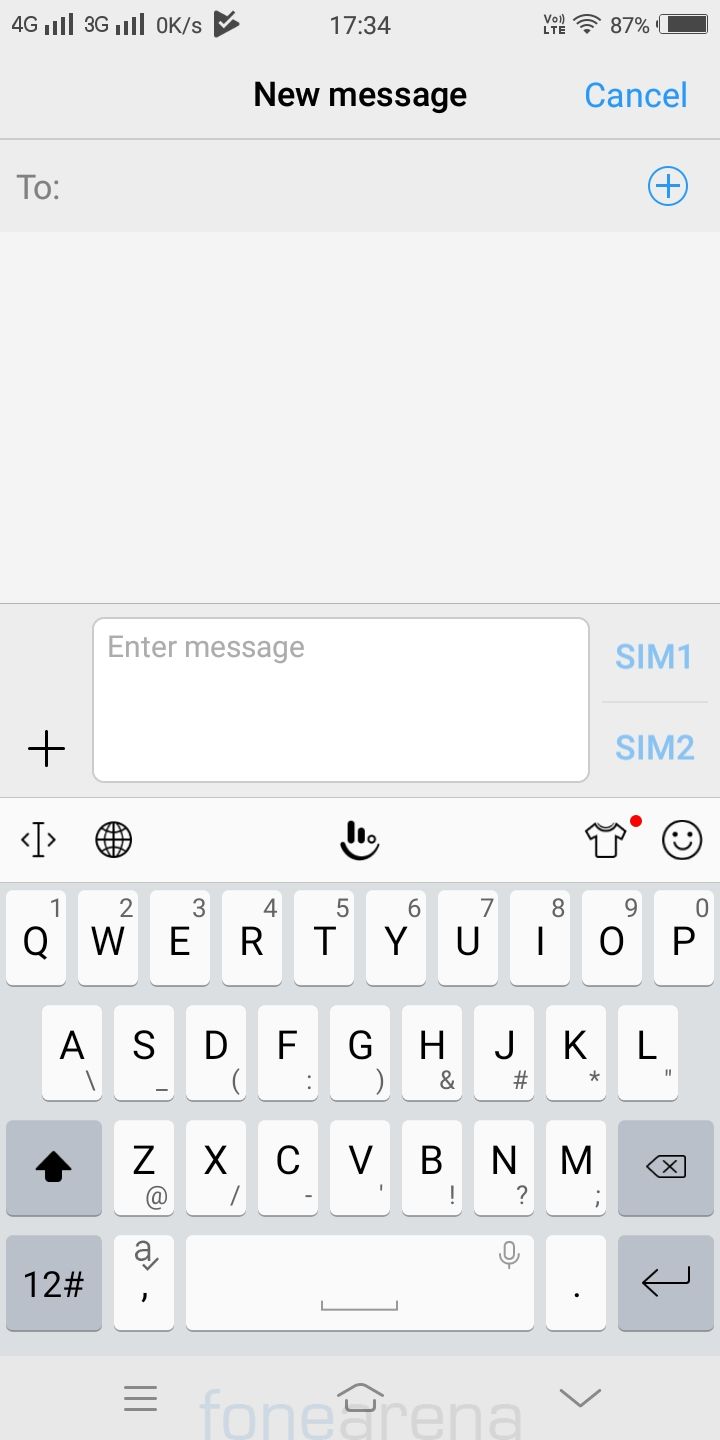The image depicts a smartphone screen with various elements. In the top left corner, it displays reception indicators showing "4G," "3G," a signal strength of "0," "K," "S," a triangle symbol, followed by numbers "17" and "34." There are two instances of "4G" and a series of Wi-Fi symbols indicating connectivity. The battery level icon reads "87%," and there's a notification for a new message. The screen also shows options labeled "blue," "cancel," and a numerical "2," accompanying a prominent plus sign. 

Within a white text input box with placeholder grey text reading "Enter message," there are two large plus signs. Additionally, the screen's status bar mentions "SIM 1" and "SIM 2," alongside an icon resembling an eye and a globe with intersecting lines. Other symbols include a connectivity bar with three bars and an icon of a shirt with a red dot in the top right corner. A smiley face is observed at the bottom section of the screen.

The on-screen QWERTY keyboard displays:
- Top row: numbers "1" to "9" and letters "QWERTYUIOP."
- Middle row: letters "ASDFGHJKL" with symbols such as slash ("/"), dash ("-"), parentheses ("()"), colon (":"), ampersand ("&"), pound ("#"), and star ("*").
- Bottom row includes: up arrow, black arrow in the middle, and letters "ZXCVBNM" ending with the backspace key.